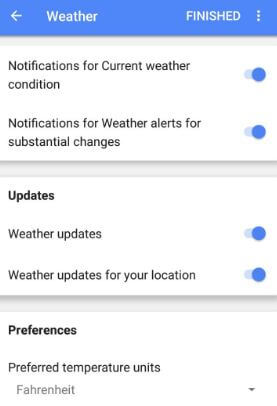This screenshot depicts an interface displaying detailed weather information settings, though it's unclear if it is from a website or an app. The interface features a distinct blue bar at the top with white text. On the far left of the bar, there is a left-pointing arrow. Proceeding to the right, the word "WEATHER" is prominently displayed in capitalized white text. On the far right, the word "FINISHED" appears in all caps, followed by a clickable three-dot menu icon.

Below the blue bar, the interface has a white background with black text. It contains several sections, each with selectable options accompanied by blue slider buttons. The options are as follows:

1. **Notifications for Current Weather Condition** - This option is turned on.
2. **Notifications for Weather Alerts for Substantial Changes** - This option is also turned on.
3. **Updates**:
   - **Weather Updates** - This option is enabled.
   - **Weather Updates for Your Location** - This option is also enabled.

The final section is labeled **Preferences**:
- **Preferred Temperature Units** - The selected unit is "Fahrenheit," which is capitalized. There is a downward arrow beside it, suggesting a dropdown menu for switching to Celsius.

This comprehensive description provides a clear understanding of the elements and settings displayed in the screenshot.